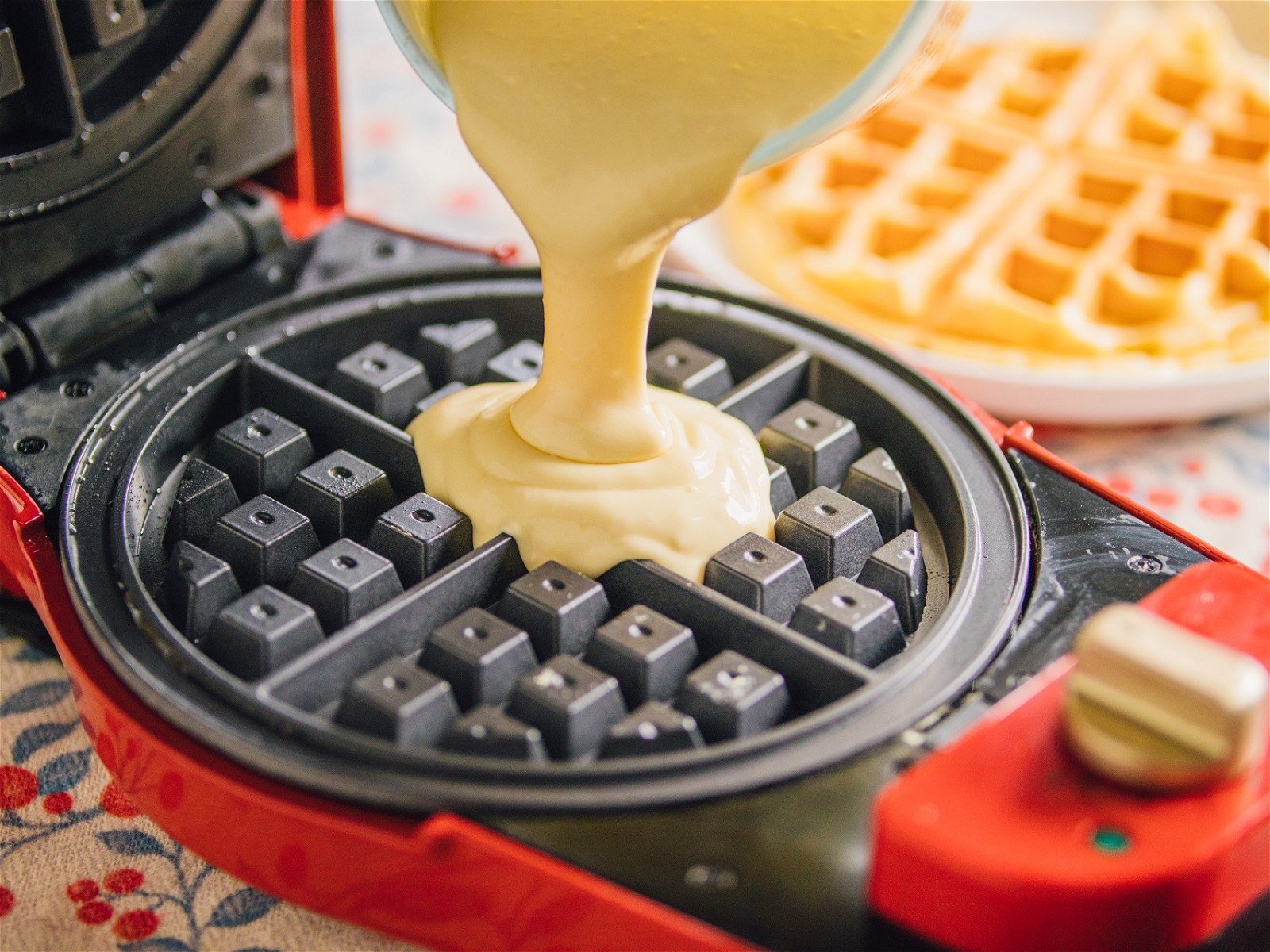In this high-resolution image, we see a red and black circular waffle maker, divided into four triangular quadrants, with a silver knob and a green indicator light on top. The waffle maker is open, revealing its black grilling surface, and is set on a table with a white tablecloth adorned with blue leaves and small red berries. In the foreground, batter is being poured from a clear measuring cup into the center of the waffle maker, only partially filling it. Off to the back right, slightly out of focus, there’s a fully cooked, golden-brown waffle resting on a plate.